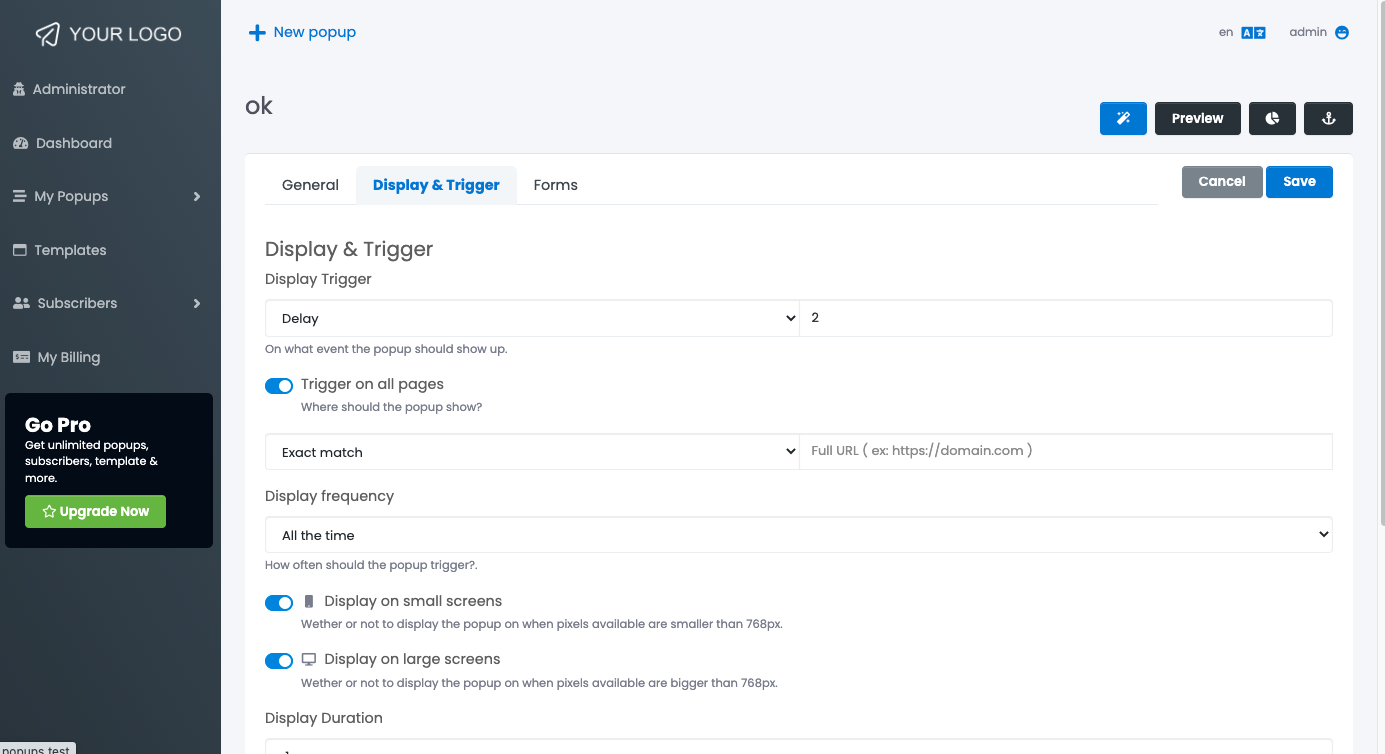At the top-left corner of the image, there is a vertically elongated, dark gray rectangle. This rectangle is fairly narrow horizontally and features the text "Your Logo" in white letters. Adjacent to this text is an upward-diagonally pointed arrow icon.

Beneath this main heading, the gray rectangle contains a series of tabs also labeled in white text. These tabs are listed as follows: Administrator, Dashboard, My Pop-Ups, Template, Subscriber, and My Billing.

Immediately below these tabs, a black rectangular box appears within the gray rectangle. This black box contains white text that reads, "GoPro: Get Unlimited Pop-Ups, Subscribers, Templates, and more." Inside the black box, there's a green rectangle featuring a star icon, followed by the text "Upgrade Now" in white letters.

To the right of the gray rectangular box, there is a blue plus sign alongside the text "New Pop-Up," followed by the word "OK." 

Underneath this section, there are three tabs labeled consecutively: General, Display & Trigger (which is highlighted in blue), and Forms. 

Further down, details under the "Display & Trigger" tab are visible. It includes the text "Display & Trigger", followed by specifics such as:
- Display Trigger Delay: 2 (displayed in a box),
- Triggers on All Pages,
- Exact Match,
- Display Frequency: All the Time,
- Display on Small Screens,
- Display on Large Screens.

These fields and labels are systematically arranged, providing a comprehensive layout of the Administrator Dashboard interface.